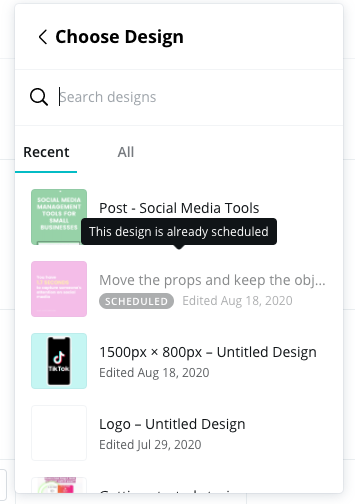This screenshot captures a section of a design-focused website interface on an all-white background with black text. 

At the top left, the header reads "Choose design," accompanied by a left-pointing arrow. Directly below, there is a search box featuring a magnifying glass icon. The search box displays placeholder text in light gray that reads, "Search designs."

Beneath the search box, two tabs are visible: "Recent" and "All," with the "Recent" tab being selected and highlighted by a blue underline. The first item under the "Recent" tab is a design labeled "Post Social Media Topics," overlaid with a notification stating, "This design already selected." 

Following that, the second recent result is titled, "Move the Props and Keep the Objects," marked as "Scheduled" but grayed out, indicating it is not currently active. This design was last edited on August 18, 2020.

The third item is "1500px by 800px, Untitled Design," also edited on August 18, 2020. The fourth and final item listed is "Logo-Untitled Design," which was last edited on July 29, 2020.

This screenshot depicts a user interface where one can search, select, and manage various design projects, highlighting the user's activity from late July to mid-August 2020.